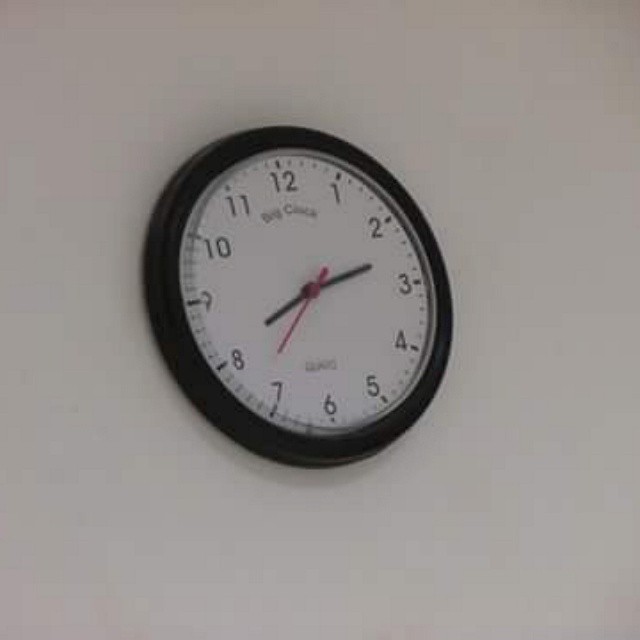A classic black clock is mounted on a stark white wall, creating a striking contrast that draws the eye. The clock face features the standard numerical markings from one to twelve, with the time precisely showing 8:13. The black minute and hour hands contrast sharply against the white background, making them easy to read. The red second hand adds a slight pop of color and is currently resting on the seventh second mark. Though the font is somewhat blurred, it appears that there may be some text on the clock face, possibly reading "Big Clock." The simplicity of the clock's design is both elegant and functional, making it a timeless addition to any space.